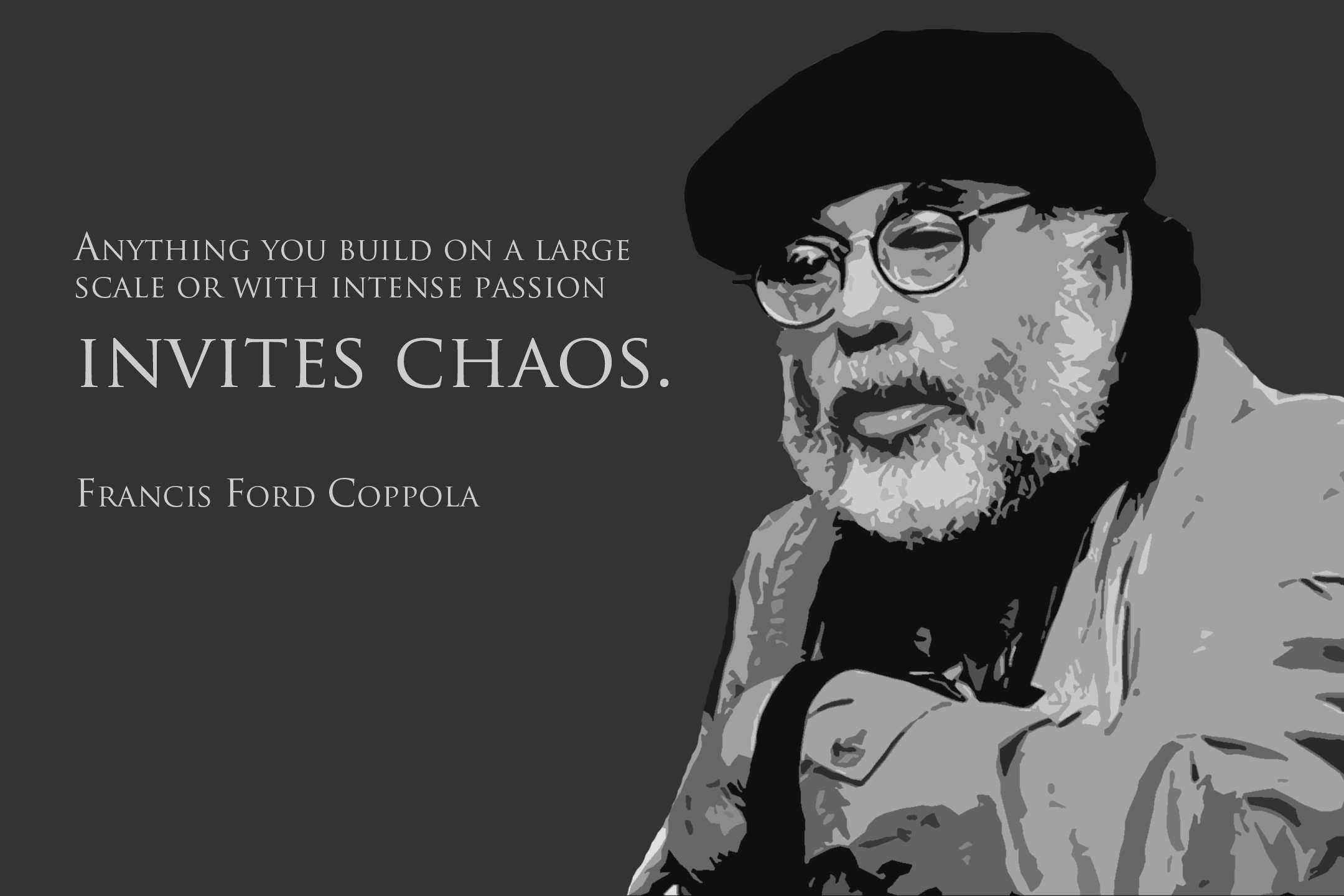The image features an abstract, sepia-toned depiction with a dark grey to black background. On the right-hand side, an elderly man, identified as Francis Ford Coppola, is prominently featured. He sports a white beard and mustache, wears a black beret, and round black-framed glasses. Coppola is dressed in a light-colored coat with a dark scarf or possibly a black garment beneath it, and his arm is bent at the elbow, suggesting a thoughtful pose. On the left-hand side of the image, a light gray text in two different font sizes stands out against the dark background. The text reads, "Anything you build on a large scale or with intense passion," followed by a larger text underneath that states, "invites chaos." Below this, in white block capital letters, it reads "FRANCIS FORD COPPOLA," identifying both the figure and the author of the quote.